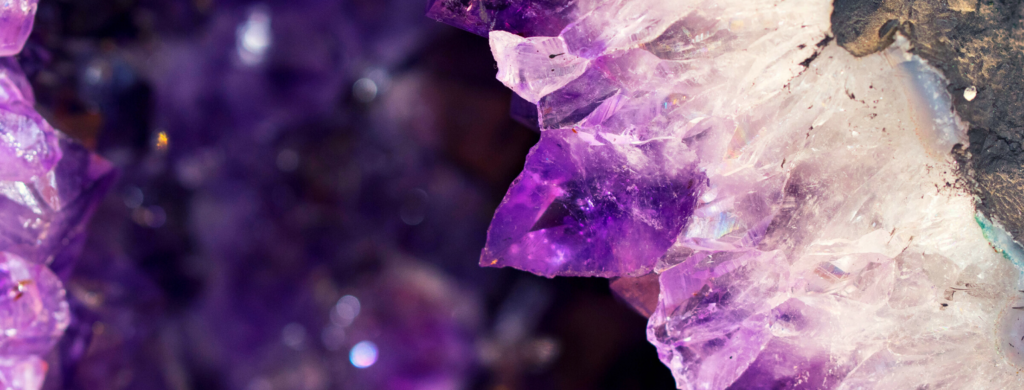This image showcases a close-up view of a striking amethyst crystal formation, prominently featuring the right side of the cluster. The amethyst crystal displays a pointed spike characterized by its dark to light purple gradient, transitioning from a deep, rich purple at the jagged peaks to a lighter hue as it merges with the white rock beneath. The upper right corner reveals a dark stone to which the amethyst is attached, adding contrast to the vibrant crystal. The blurred background enhances the glistening spots and darker shades of purple, providing a shimmering effect across the photo. On the far left, the image captures a segment of another amethyst formation, characterized by its lighter, translucent purple. The overall composition of the photo, laid out horizontally, accentuates the intricate details and natural beauty of the amethyst, from its crystalline spikes to the textured geode-like exterior.